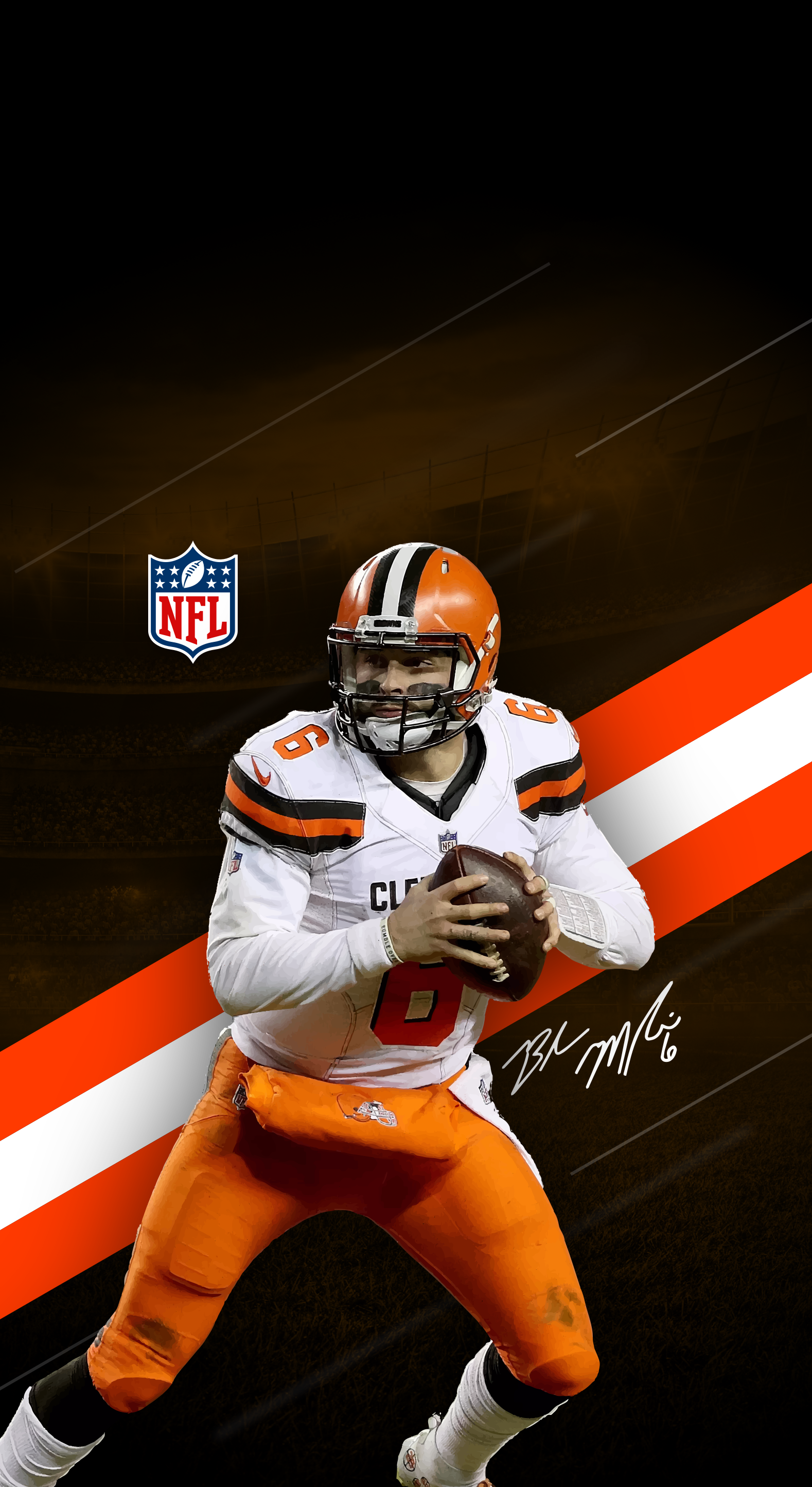This image features a detailed and signed poster or card of Baker Mayfield, the NFL quarterback. Dominating the center, Mayfield, in full motion as if about to throw a football, is captured in his Cleveland Browns uniform. His distinctive gear includes a white jersey with orange and black stripes, sporting the number six on both the front and shoulders, accompanied by burnt orange pants and an orange helmet. The background showcases a deep brown color with diagonal orange and white stripes, and a silhouette of a football stadium adds depth to the scene. Hovering above Mayfield's right shoulder is the NFL logo, while just below him lies his signature. The overall image adopts a black, brown, white, blue, red, orange, and gray color palette, and comes together as a collectible sports souvenir.